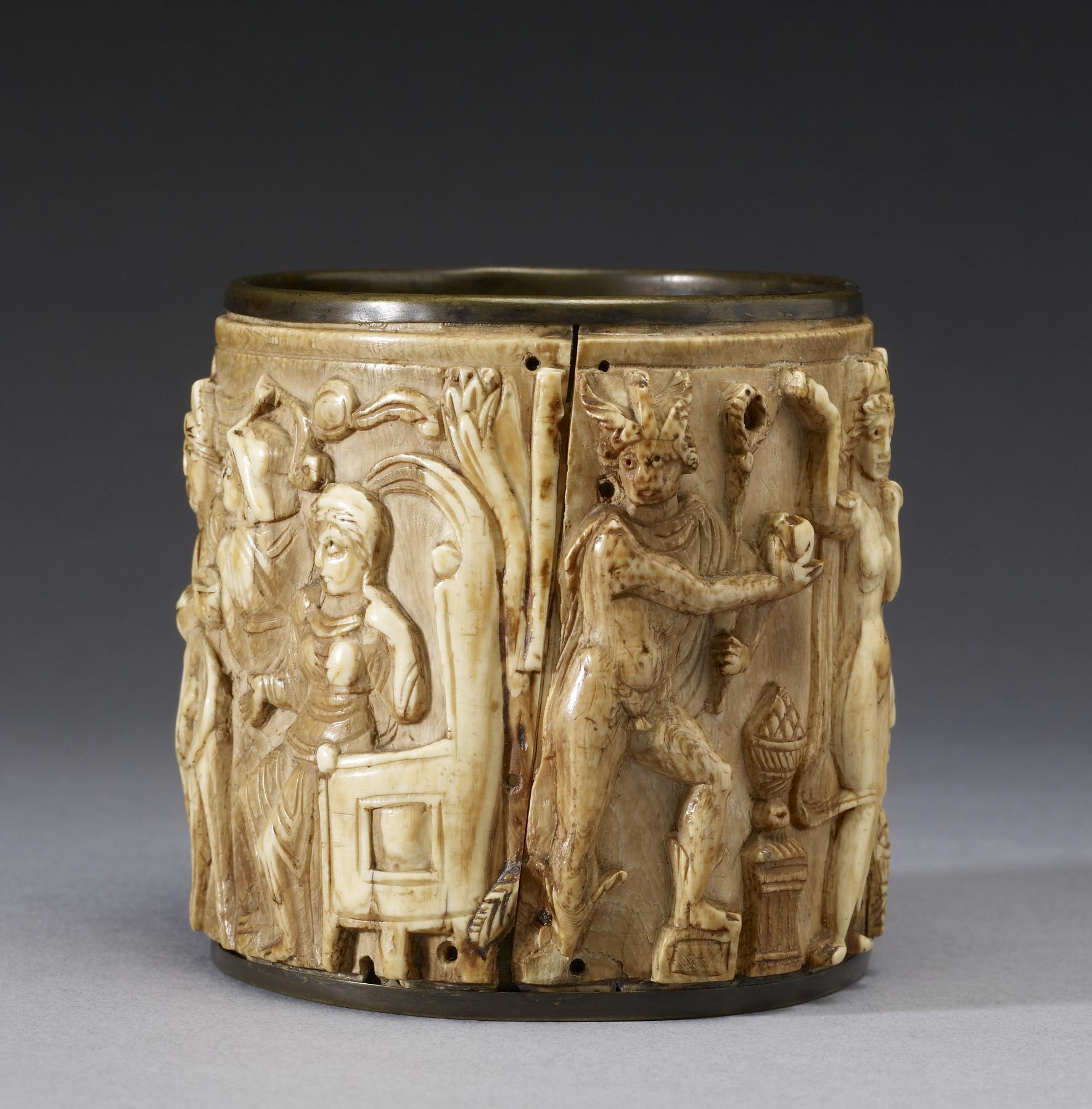The photograph depicts a meticulously crafted ancient relic that resembles a container, possibly a cup or mug, though it notably lacks a handle. The vessel is adorned with intricate carvings that encircle its entire surface. These carvings feature human figures and a potentially regal or ceremonial scene. Notably, the artwork includes a man holding a staff and wearing a headdress, possibly of Mesoamerican or Egyptian influence, and a naked woman seated on a throne. The carvings are lighter brown, contrasting with the dark brown top of the vessel. The material remains uncertain, possibly ivory, wood, or ceramic, with its color ranging from light to medium brown. The relic rests on a gray surface that could be a table or floor, suggesting that the item is displayed for viewing or sale.